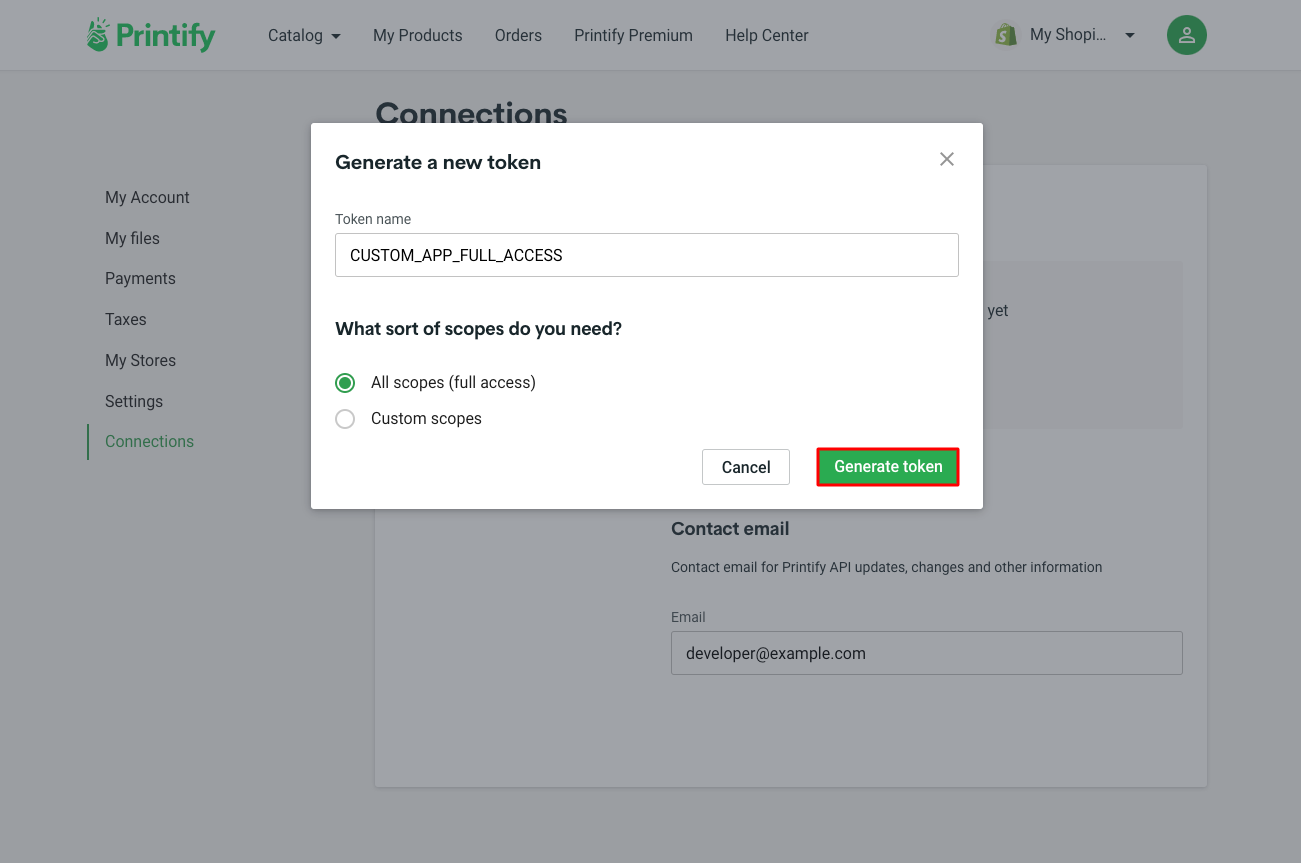The image features a user interface from Printify, prominently set against a gray background. In the upper left corner, displayed in green text, is the word "Printify." To the right of this, there are several menu options, listed sequentially: "Catalog," "My Products," "Orders," "Printify Premium," and "Help Center."

On the far right side of the top menu bar, there is an image of a green bag adorned with a dollar sign, next to which is the label "My Shop" accompanied by a downward-pointing arrow. Adjacent to this is a green circle containing the silhouette of a person in white, indicative of user profile settings.

Centrally positioned within the image is a white rectangle. At its top, there is a header that reads, "Generate a New Token." Below this header, the interface prompts "Token Name," followed by a search box labeled "Custom App Full Access." Beneath this, there is a query: "What Sort of Scopes Do You Need?" Next to this question is a green circle with the text "All Scopes" and the note "(Full Access)" in parentheses. Further down, there is another option titled "Custom Scopes."

At the bottom right of the white rectangle are two clickable buttons: "Cancel" on the far right, and to its left, a green square outlined in red containing the text "Generate Token."

Down the left side of the main interface area, set in a shaded sidebar, there are a series of options listed vertically: "My Account," "My Files," "Payments," "Taxes," "My Stores," and "Settings." Separating these options from the next section is a short green vertical line beside which is the word "Connections."